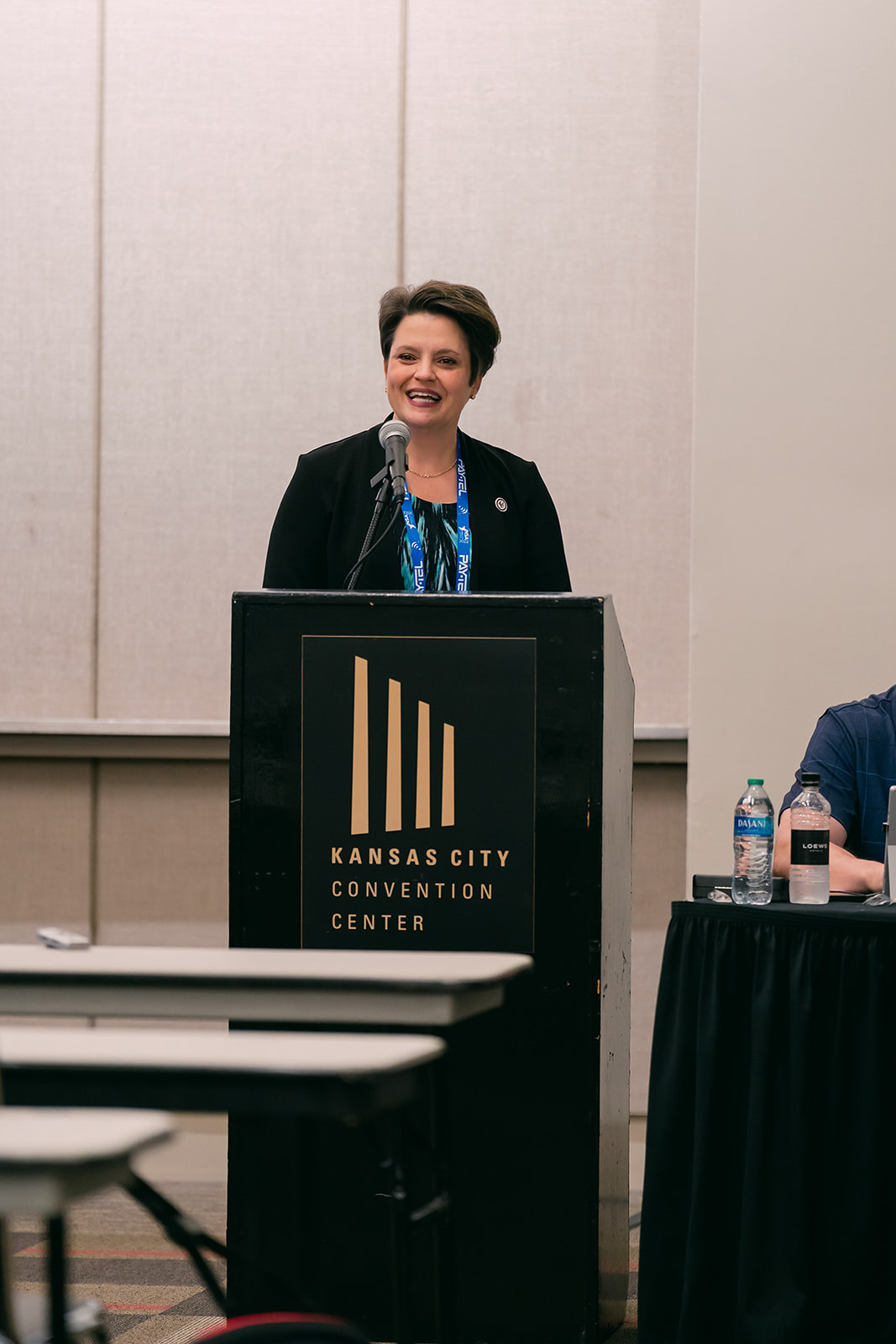The photograph captures an older white woman, likely in her 50s or 60s, delivering a speech behind a black podium equipped with a microphone. The podium bears a black sign with gold text reading "Kansas City Convention Center," adorned with a descending line pattern possibly representing buildings. She has short, dark brown hair and wears a black suit jacket over a blue blouse, accessorized with a blue identification tag around her neck. She's standing in a white convention hall, smiling as she speaks. To her left and right, folding white tables can be seen, with an arm of a panelist on her right visible, along with two water bottles. The setting suggests a formal convention environment with additional tables set up for attendees.